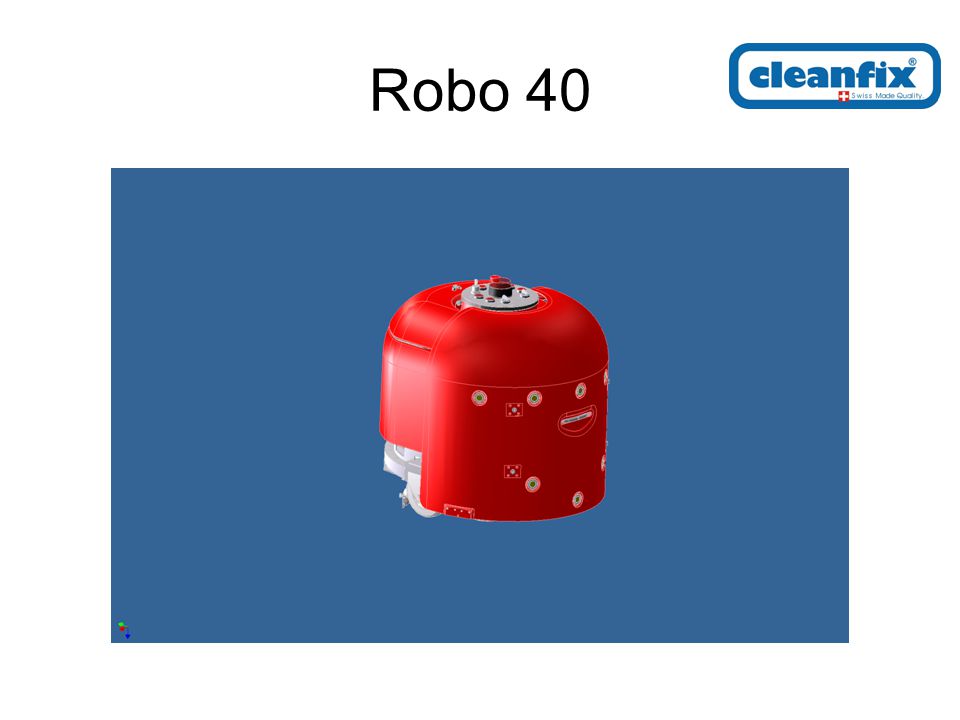The image depicts an ad for the CleanFix ROBO-40, prominently featuring both the product and branding elements. The product, which measures approximately 10 by 8 units, slightly wider than it is tall, is positioned centrally and presented in a rich red color. It has a unique design—resembling a cylinder that might have originated from a rectangle with a domed top. This gives it a helmet-like or electric motor appearance. The dome's apex showcases a distinct round, silver patch held together with bolts, potentially an access point, from which a hollow black tube emerges.

On the top right corner of the image, a blue oval rectangle carries the CleanFix branding, adorned with the text "Swiss Made Quality" and a Swiss flag emblem, accentuating its origins. Just beneath this, in bold black letters, is "ROBO-40."

Notably, the product features several sensors on its front fascia, some circular and others square, and hosts various stickers and a possible serial number. The left side reveals barely-visible wheels, suggesting the product is a mobile robot. There are also little buttons scattered on top and white plastic components protruding from the back, adding to its complex design.